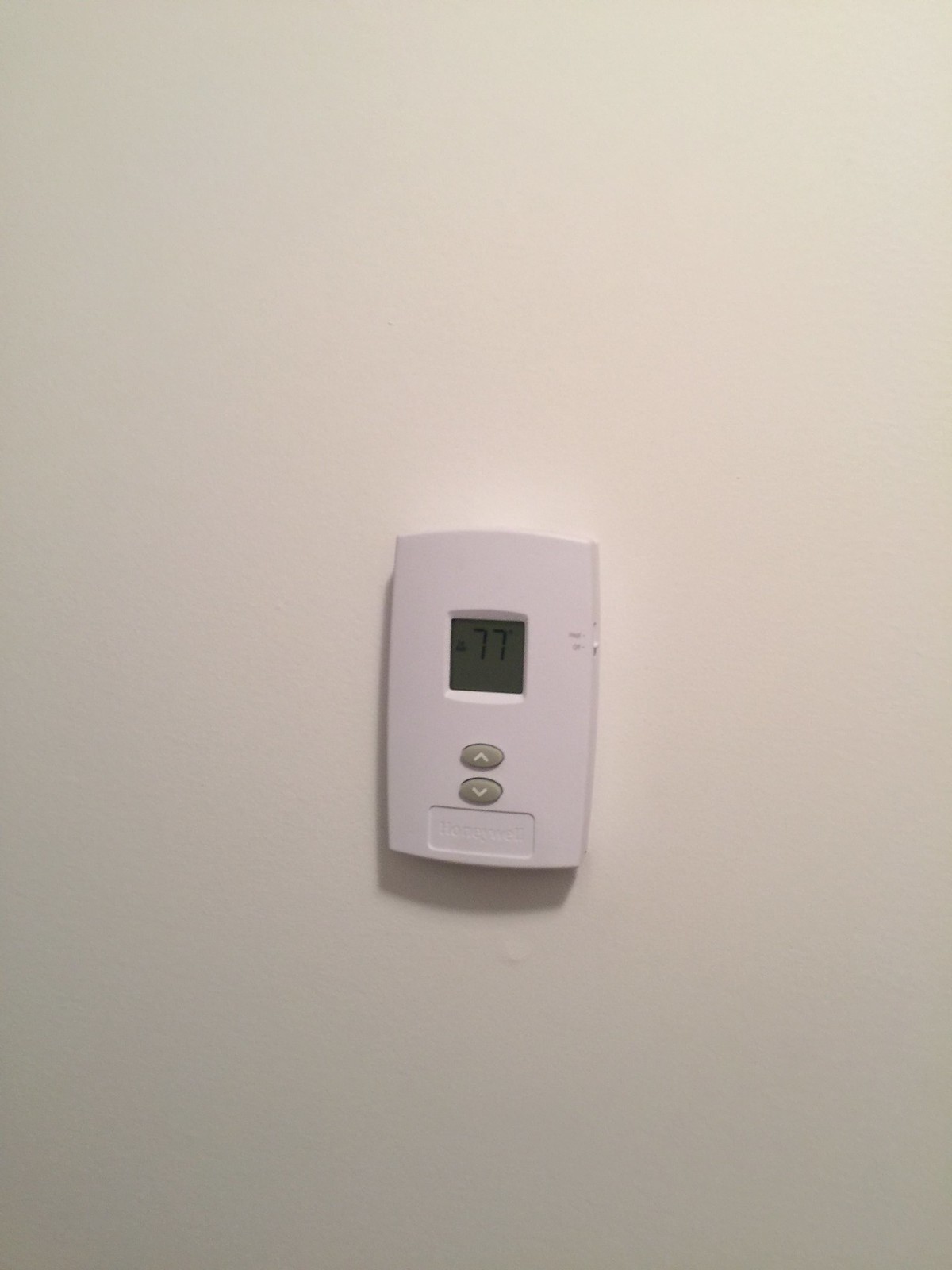The image showcases a white thermostat mounted on a plain white wall, possibly situated in a hallway, living room, or another area of a home. The rectangular thermostat features two gray circular buttons stacked vertically; the upper button has an arrow pointing upwards, while the lower button has an arrow directed downwards. On the thermostat box, there is also a distinct, textured rectangular area that appears to be a battery compartment cover, suggesting it might be pulled down for battery replacement.

A small digital display on the thermostat prominently reads "77°F," indicating the current temperature inside the home. Adjacent to the display is a small slider switch labeled with options, likely for heating, off, and cooling modes, although only two of the labels are visible and legible in the image. The thermostat casts a subtle shadow on the pristine white wall, adding a slight depth to the scene. It is unclear whether the device itself functions as a thermostat or merely a temperature reader.